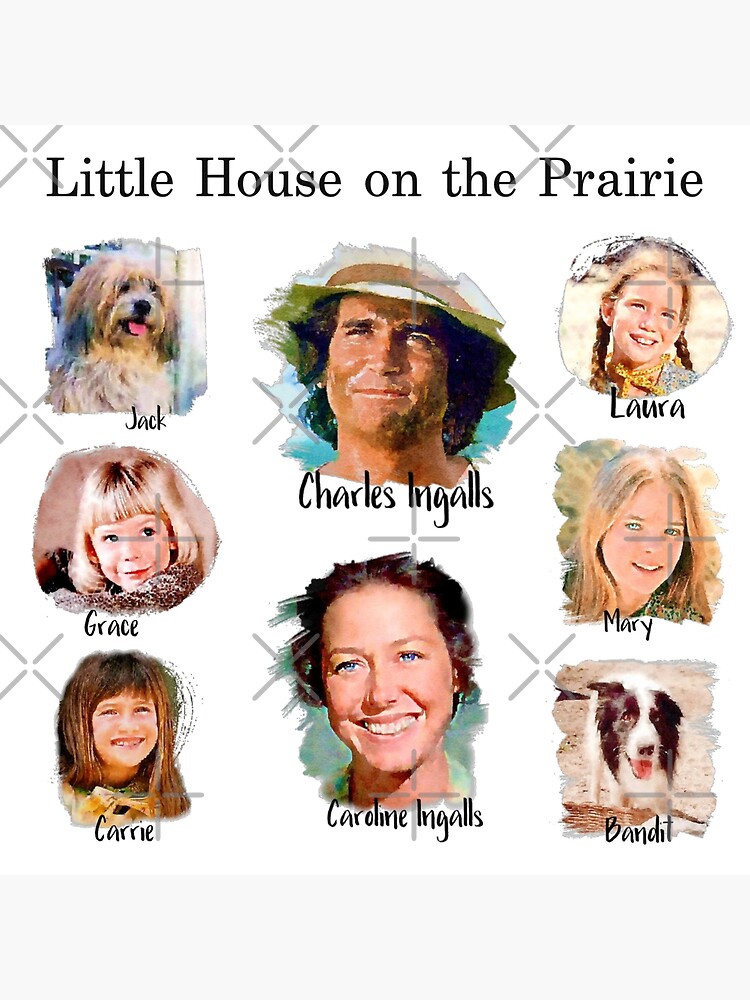This detailed poster of "Little House on the Prairie" showcases a collection of characters from the show against a white background with a diamond plate-like texture behind them. At the center of the poster is Charles Ingalls, a middle-aged man with brown shoulder-length hair and a sun hat, and Caroline Ingalls, his wife, who has short brown hair and deep blue eyes, both smiling. The left column features Jack, a shaggy dog with a predominantly white fur coat and distinctive brown and blue markings on its face and ears; Grace, a young blonde girl with a crown of darker blonde hair, wearing a brown shirt; and Carrie, a smiling girl with shoulder-length brown hair and brown eyes. The right column includes Laura, a girl with brown pigtails and a yellow-orange bow tie, wearing a greenish-blue floral dress; Mary, a girl with blonde hair, greenish-blue eyes, and a green dress with red floral accents; and Bandit, a white dog with brown ears and a large brown spot on the left side of its face, set against a background of brown dirt. The title "Little House on the Prairie" crowns this charming ensemble, reflecting the wholesome essence of the beloved characters of the show.